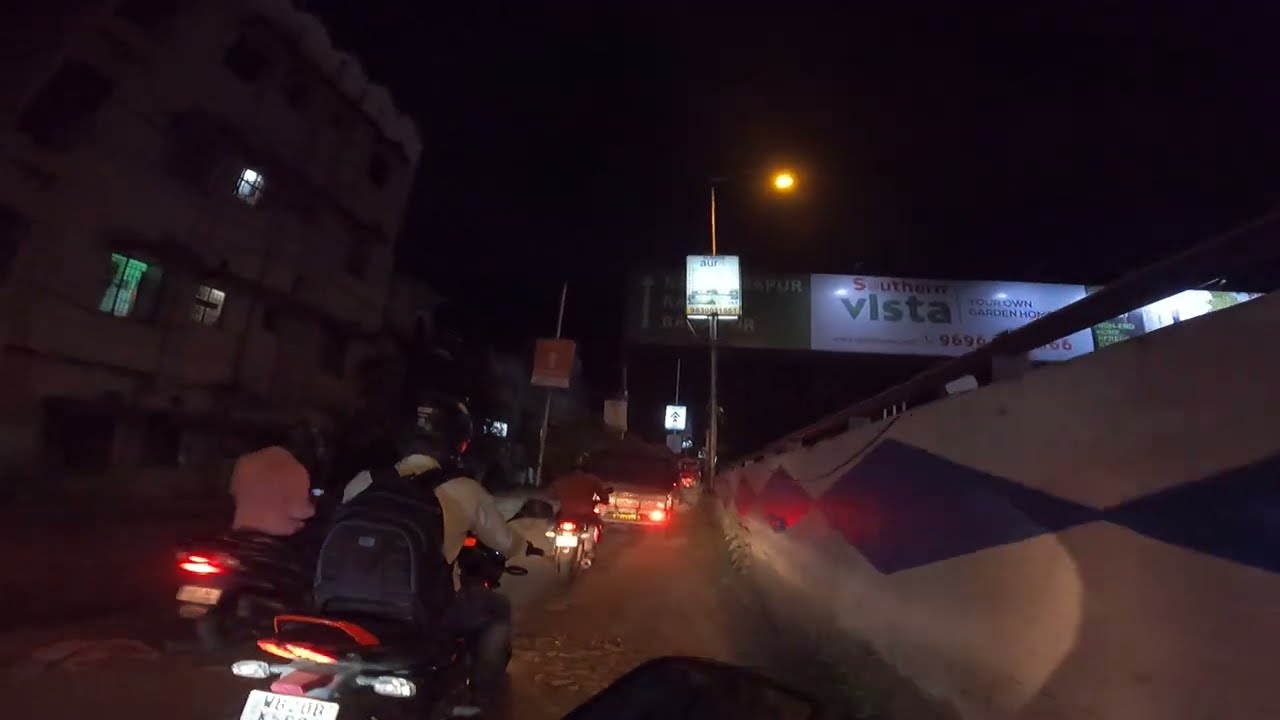This nighttime urban scene is viewed from the perspective of a biker on a congested city road. The camera reveals the small front portion of the bike. Directly ahead, two individuals are riding scooters or mopeds. The closer rider, positioned slightly to the front left of the viewpoint, is wearing a backpack and a black helmet, paired with a white shirt and grayish pants. Another rider, slightly farther left, sports a white top and dark pants. In front of them are several other vehicles, both bikes and cars, their headlights piercing the darkness.

To the left, a four to five-story residential concrete building has several lit windows, adding a warm glow to the scene. This building likely serves as an apartment complex. On the right side of the road, there is a distinctive concrete wall adorned with a blue diamond pattern and topped with a railing, alongside a boundary painted white and blue. Overhead, a yellow streetlight illuminates the area, casting a soft glow on the vehicles below.

The road is lined with various signage, including street signs and billboards. In the distance, a prominent billboard with the words "Southern Vista" and "Your Own Garden" stands out, although some other text is not clearly visible. Additionally, there are several poles supporting smaller boards. A concrete bridge or ramp is also noticeable in the background, enhancing the depth of the urban scenery. The entire scene is under a black, night sky, accentuated by the various light sources from vehicles and streetlights.